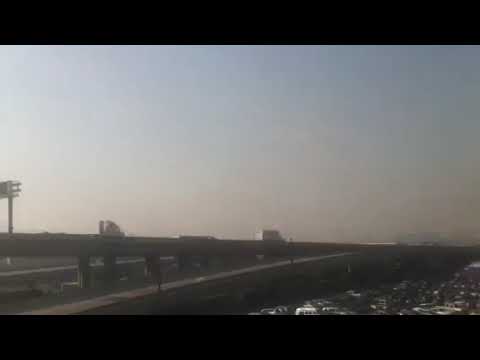In this outdoor photograph, taken on a very hazy and foggy day, there is a distant view of a freeway winding through the scene. The picture, though blurry, captures the gray, overcast sky which dominates the backdrop. The freeway itself, a dark, prominent line, is depicted with two roads leading from the left to the center of the image, bordered by trees and a green median. The far distance reveals one or two buildings faintly standing above the landscape. In the lower part of the image, particularly on the right, there is a cluttered parking lot with numerous vehicles, mostly black and a few white, appearing tiny and indistinct due to the haziness. On the left side of the picture, a large street light stands out, potentially illuminating the area during the night. There is also a path leading up to the main road, possibly with a bus or an open window vehicle moving along it.